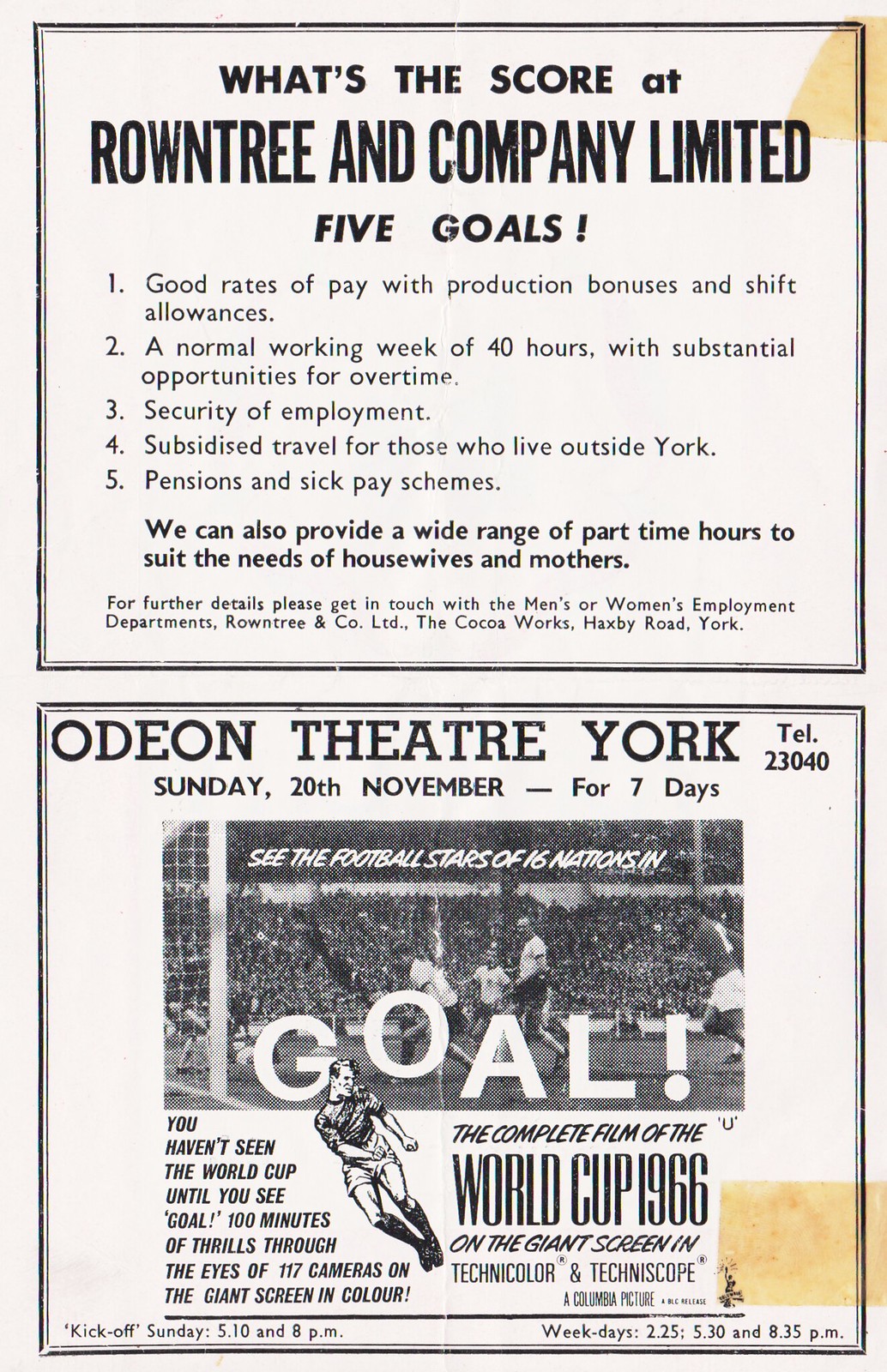This is an image of a vintage-style pamphlet, featuring two distinct sections separated by a black border. The top section serves as an advertisement for Roundtree and Company Limited, titled "What's the score at Roundtree and Company Limited? Five Goals". It lists five key benefits offered by the company: good rates of pay with production bonuses and shift allowances, a 40-hour working week with substantial overtime opportunities, employment security, subsidized travel for employees living outside York, and comprehensive pensions and sick pay schemes. Additionally, the company offers a variety of part-time hours to accommodate housewives and mothers. For further details, it provides contact information for their Men's and Women's Employment Department located at The Cocoa Works, Haxby Road, York. The background is a pink paper, evoking the feel of an old magazine page.

The bottom section promotes a show at the Odeon Theatre in York, advertising the screening of the complete film of the 1966 World Cup titled "Goal". It details that the movie will be shown on Sunday, 20th November, for seven days, and highlights the unique experience of watching 100 minutes of thrilling football action through the eyes of 117 cameras, showcased in full color on a giant screen using Technicolor and Techniscope. There is an image depicting a football field with players, reinforcing the energetic and immersive viewing experience being offered.